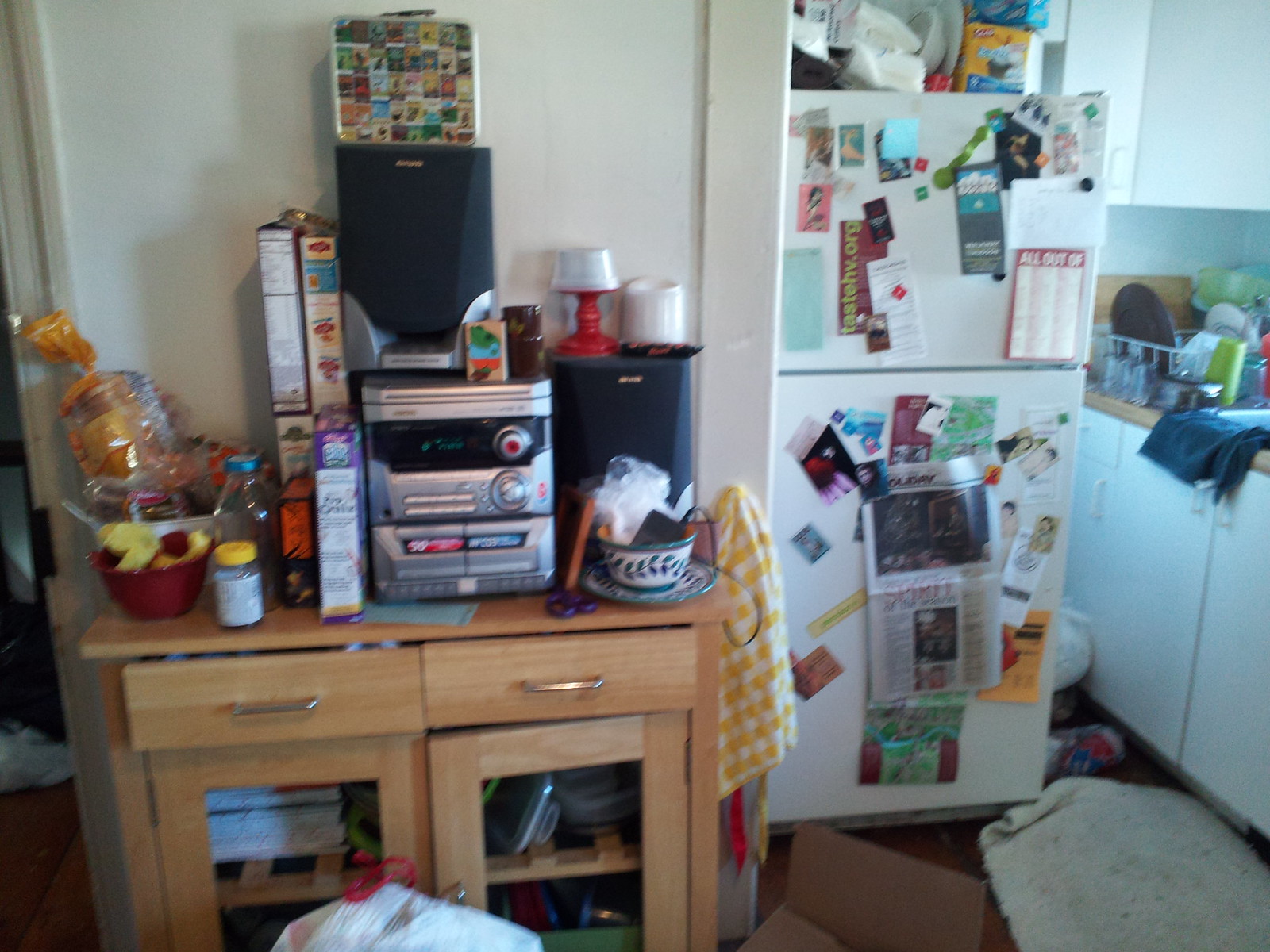The image depicts an extremely cluttered kitchen, reminiscent of an efficiency apartment due to the multitude of items scattered throughout the space. On the right side, there is a white refrigerator, heavily adorned with a variety of colorful magnets and newspaper clippings, featuring hues such as gray, white, black, red, green, and yellow. Atop the refrigerator sits an assortment of items, adding to the overall disarray.

Next to the refrigerator is a white kitchen cabinet, above which a white wire dish rack holds a large, round, brown dish. On the countertop, which appears to be a light brown color, lies a blue cloth. The kitchen cabinetry, both upper and lower, is uniformly white.

On the left side of the image, a brown wooden cabinet stands. It features two wooden glass doors and two partially open drawers. Atop this cabinet, a silver and black stereo system is placed, flanked by matching silver and black speakers—one on top of the stereo and the other to its right. Nearby, several cereal boxes are visible, though their brands are indiscernible. Leaning against the white wall to the left of the cabinet is a loaf of bread in its packaging. Additionally, a bottle with a white label and a yellow cap is visible, and beside it sits a red bowl containing something yellow. A white garbage bag with red plastic ties rests against the wooden cabinet. The image contains no readable text.